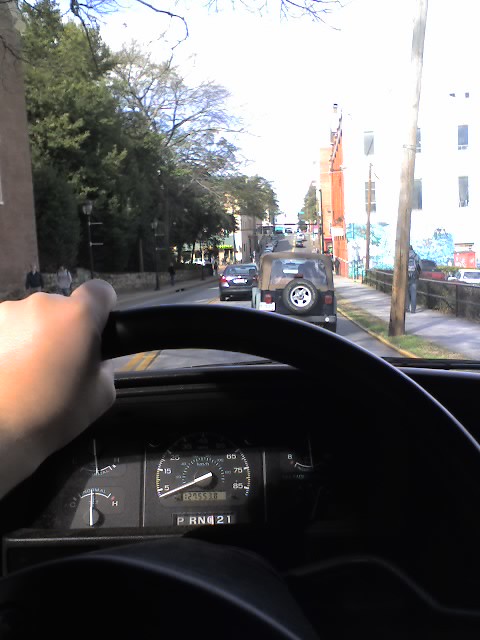The image, captured from the driver's perspective, shows a stationary vehicle with the speedometer indicating zero. The driver’s left hand is gripping the top of the steering wheel, while their right hand appears to be taking the photo. The interior suggests an older vehicle, characterized by its manual dials. The view ahead reveals a two-lane road, one lane in each direction, with cars lined up at a traffic light. To the left, leafy trees line the street, while on the right, various buildings suggest an urban or city setting. Pedestrians can be seen walking on both sides of the street, adding to the urban atmosphere.